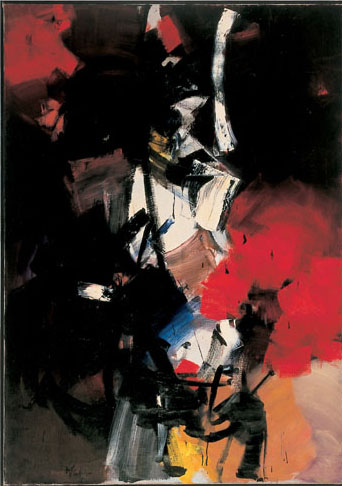This image showcases a striking piece of abstract artwork, predominantly characterized by deep black hues interwoven with vibrant colors. The composition features extensive dark black areas, especially on the left side and the upper corners, contrasted sharply by bright red patches to the right and upper left. A central section of the painting is highlighted by white, with additional splashes of yellow and tan towards the bottom middle. The artwork also incorporates blue, orange, and gray tones, creating a visually cluttered and layered effect that evokes different interpretations from each viewer. There are no discernible objects or text, as the painting seems to be a complex interplay of overlapping shapes and colors, forming an intricate, multi-layered structure. This detailed and distinctive piece likely reflects personal or artistic expression and would not seem out of place hanging in someone's home.